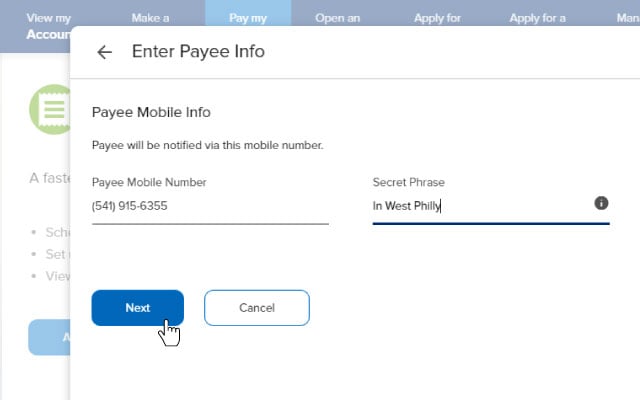In the image, a pop-up window dominates the foreground, obstructing some content in the background. This secondary layer of information features a light blue header with a "View My Account" tab visible on the top left, complemented by several partially obscured tabs with white text. The main background is predominantly white, featuring a blue button situated in its bottom left corner.

Shifting focus to the pop-up window in the foreground, the interface sports a clean white background with black text. Positioned prominently in the top left corner is the title "Enter Payee Info." Below this heading, the section "Payee Mobile Info" requests a mobile number for notifications, already filled in with the number 541-915-6355. Adjacent to this is a field labeled "Secret Phrase," which displays the phrase "In West Philly."

The bottom left corner of the pop-up window showcases two action buttons: a blue "Next" button and a "Cancel" button outlined in blue. A cursor, represented by a pointing finger, is hovering over the "Next" button, indicating the user's intention to proceed.